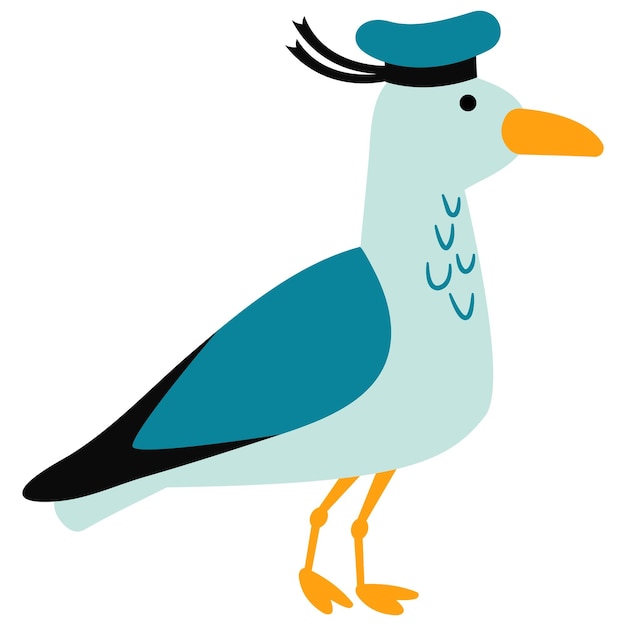This detailed computer cartoon illustration features a whimsical seagull standing against a white background. The seagull, predominantly light blue, dons a dark blue sailor's hat adorned with black rims and two flowing black ribbons. The bird’s eyes are black, and it sports a distinctive yellow beak. Underneath the beak, you can find five darker blue U-shaped markings along its neck. Its prominent wing, matching the dark blue of its hat, is tipped with black. The bird’s two yellow, webbed feet with notably bent knees provide support below its light blue underbelly. The bird faces left, creating a dynamic and playful stance in the simplistic, unobstructed setting.